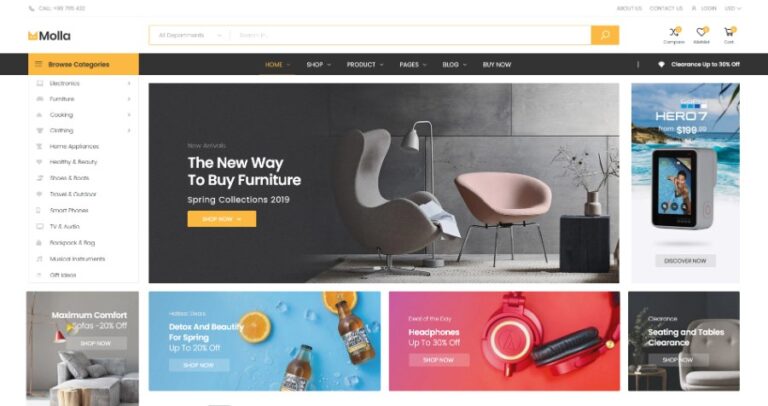The webpage features a visually engaging layout with the brand name "MOLA" prominently displayed at the top. Below the brand name is a search box labeled "All Departments," accompanied by a bright orange search button on the right. To the left, users can explore various categories such as Cooking, Furniture, Home Appliances, Health & Beauty, TV & Audio, and Smart Homes, although some categories are not fully visible.

In the center of the page, a bold, white text against a black background reads, "Review Awards: The New Way to Buy Furniture, Spring Collection 2019." Just below this header is an orange "Buy Now" button. Adjacent to this central message are product displays, including a gray couch, a pink chair, and a black speaker adorned with a green plant. The walls surrounding these items are gray, adding a modern touch to the décor.

On the right side of the page, a promotional section advertises the Hero 7 video camera for $199.99. Below, a vibrant banner announces the "Maximum Comfort Sale" with a 20% discount and a "Shop Now" call-to-action button. Additional offers including "Detox and Beauty for Spring - Up to 20% Off" and "Headphones - Up to 30% Off" are displayed with colored backgrounds; blue for detox and pink for headphones, each with their respective "Shop Now" buttons.